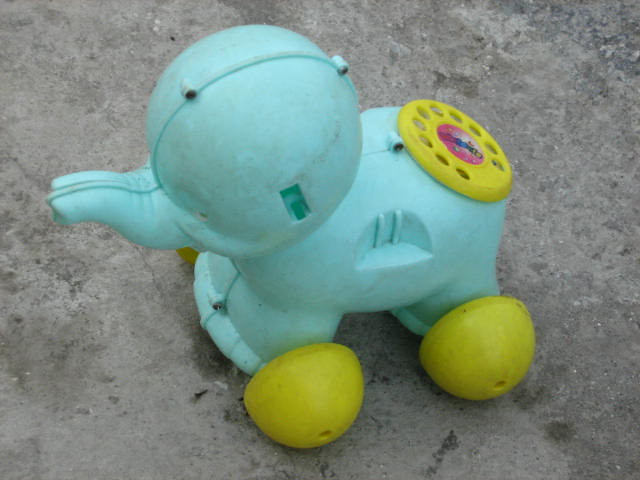This is a square, close-up photographic image taken outdoors during the day, depicting a well-worn and dirty child's toy. The toy, a light blue plastic elephant with a large head and small trunk, is positioned diagonally and centered on an old, stained concrete surface. The elephant features a distinct seam running through the middle of its head, indicating the presence of hinges. Instead of a tail, the back of the toy is equipped with an old-style rotary dial reminiscent of vintage telephones, featuring a pink circular center. Its wheels are large and yellow. The concrete background is marked with dark gray stains, adding to the overall sense of age and wear. The absence of text in the image further emphasizes the focus on the toy elephant and its nostalgic, albeit dilapidated, condition.